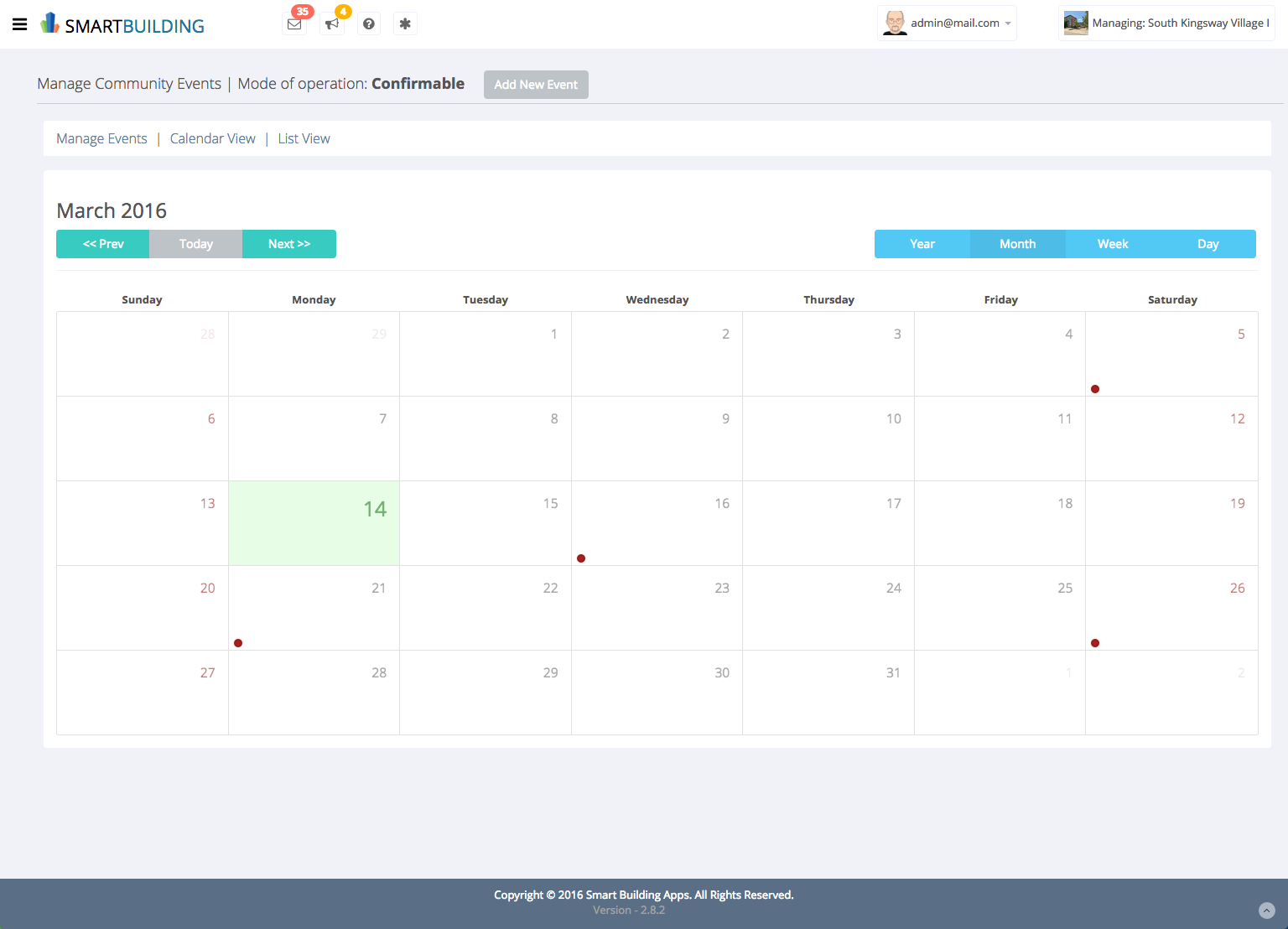A detailed website screenshot displays the interface of a Smart Building management application. In the top left corner, the title "Smart Building" is prominently featured. Adjacent to the title, there are four icons: an email icon with a red notification indicating '35' unread messages, a megaphone icon with '4' notifications, a question mark icon possibly serving as a help or FAQ link, and an asterisk icon, likely used for additional settings or options. 

At the top right corner, there is a cartoon avatar of a white man, labeled with the email "admin@mail.com." Beside this avatar, a small, blurry photograph of a building is displayed along with the text "Managing South Kingsway Village 1." Below this, there are multiple actionable buttons for managing various features: "Manage Community Events," "Mode of Operation Confirmable," "Add New Event," "Manage Events," and options for viewing the calendar in "Calendar View" or "List View." 

The calendar showcased is set to March 2016, offering navigation buttons labeled "Previous," "Today" (which is selected), and "Next." To the right of these, options for viewing the calendar by "Year," "Month," "Week," or "Day" are available. The month layout spans from Sunday to Saturday, starting with Tuesday as the first day of March and ending with Thursday as its last day. Several dates are highlighted with red circles, specifically on Saturday, March 5th; Saturday, March 12th; Wednesday, March 16th; Monday, March 21st; and Saturday, March 26th. March 14th is highlighted in light green, indicating a special status or event. 

At the bottom of the screenshot, there is a footer displaying "Copyright 2016, Smart Building Apps, All Rights Reserved," and the software version "Version 2.8.2."